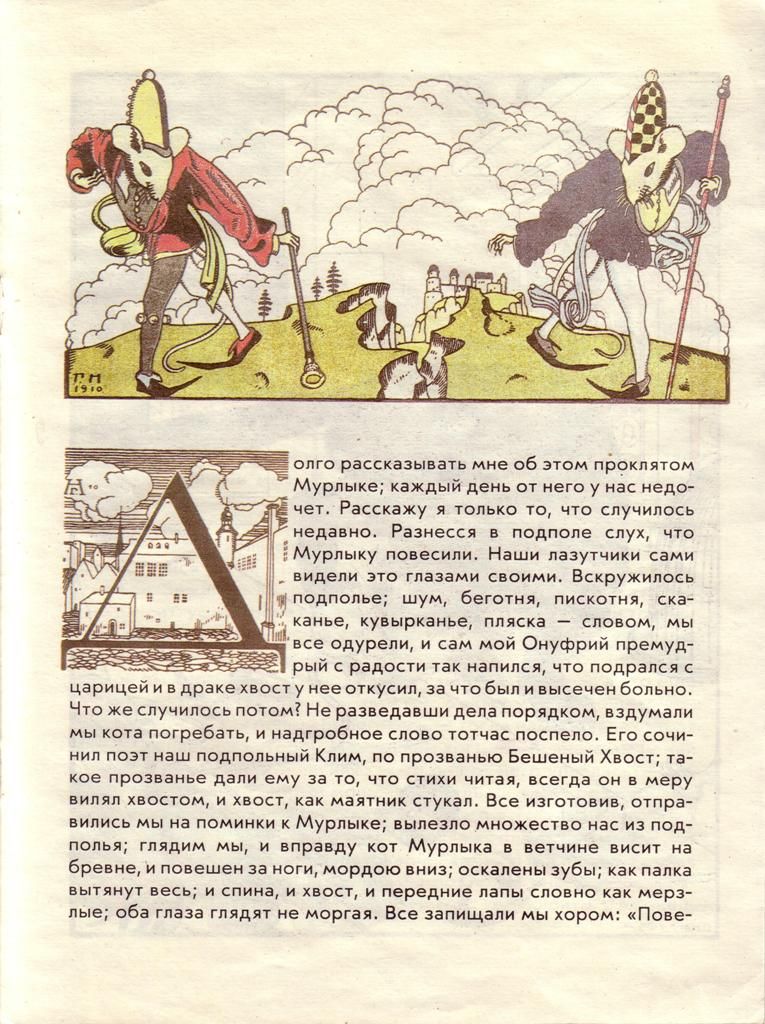The scanned image presents a yellowed page from an aged book. The top section features an intricate illustration depicting two human-like rats standing on opposite sides of a cliff covered in green grass, looking at each other. The rat on the left is adorned in a red coat with gray hose and red and black shoes, holding a scepter ending in a suction cup. The rat on the right dons a blue coat with white hose and gray and black shoes, and carries a long stick. Both rats are dressed in ornate, medieval puffy-sleeved costumes and tall, thin, rounded hats, with one leg forward as if mid-step or dance, and arms outstretched towards each other. Deep in the background, a castle sits atop a distant hill, with large, puffy white clouds overhead. The bottom half of the page is densely filled with black text in Cyrillic script, starting with a large, ornate letter 'A'.